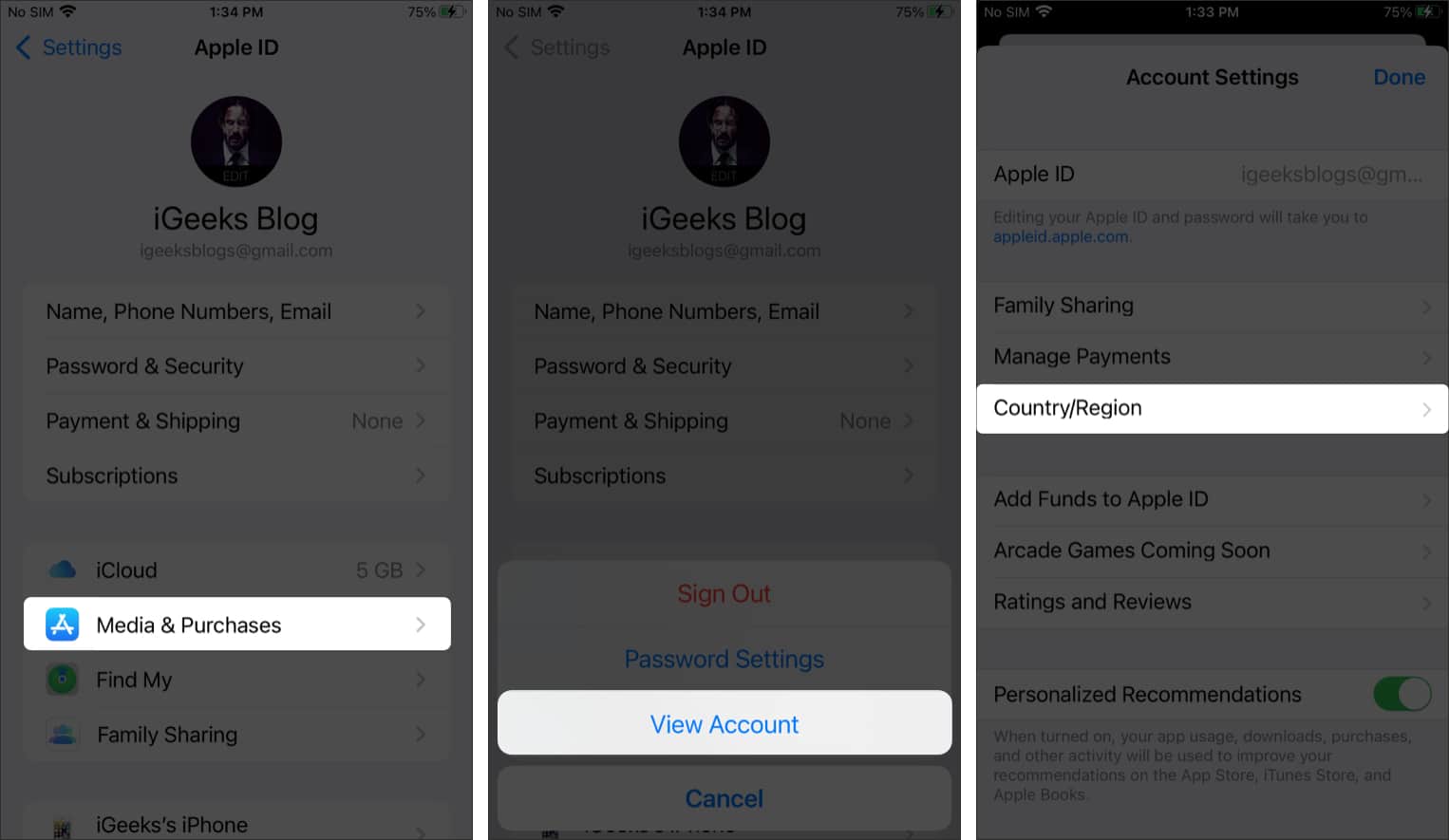This image displays three smartphone screens each presenting segments of various account settings. 

On the leftmost screen, most sections are grayed out except for “Media & Purchases.” The middle screen shows an "Account" page with an option labeled “View Account” that stands out as not grayed out. The rightmost screen displays options for "Country/Region" also not grayed out. 

Below all three screens, a list of account-related options is visible:
- Name, phone number, email
- Password & Security
- Payment & Shipping
- Subscriptions
- iCloud
- Media & Purchases
- Find My
- Family Sharing

Additional details visible on the screens include:
- The middle screen lists “Sign Out” in red, with “View Account” and “Cancel” in blue.
- The rightmost screen features "Account Settings" with a blue "Done" button below it. Underneath, it shows an Apple ID associated with "iGeeksBlog@gmail.com," along with an "Edit" prompt which redirects to appleid.apple.com for further modifications.

This image appears to be a guide to navigating through different important settings linked with an Apple ID on an iPhone.